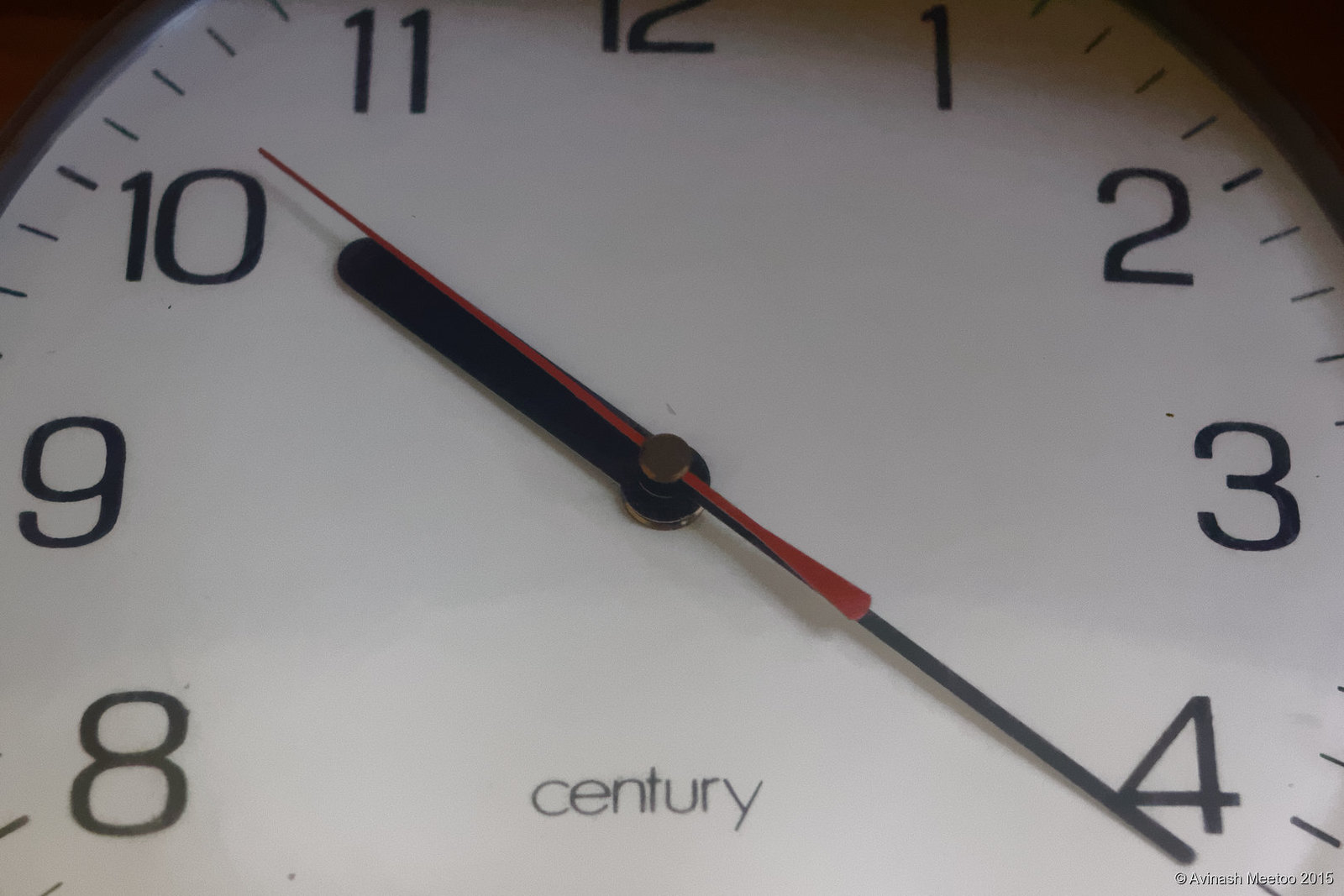This is an extreme close-up image of an analog clock lying face-up on a medium-toned wooden surface. The wooden surface is visible in the top left and right corners of the image, framing the clock. The visible portion of the clock reveals about two-thirds of its face, displaying the numbers 1 through 4 on the right side and 8 through 11 on the left, with a partial view of the number 12 at the top. Minute markers, including tiny lines next to each number and additional lines between them, indicate intervals, likely every two minutes.

The clock features three hands: an hour hand, a minute hand, and a second hand. The hour hand points slightly past the 10, the minute hand is just after the 4, and the second hand is just after the 10. The time displayed on the clock is approximately 10:22 and 54 seconds.